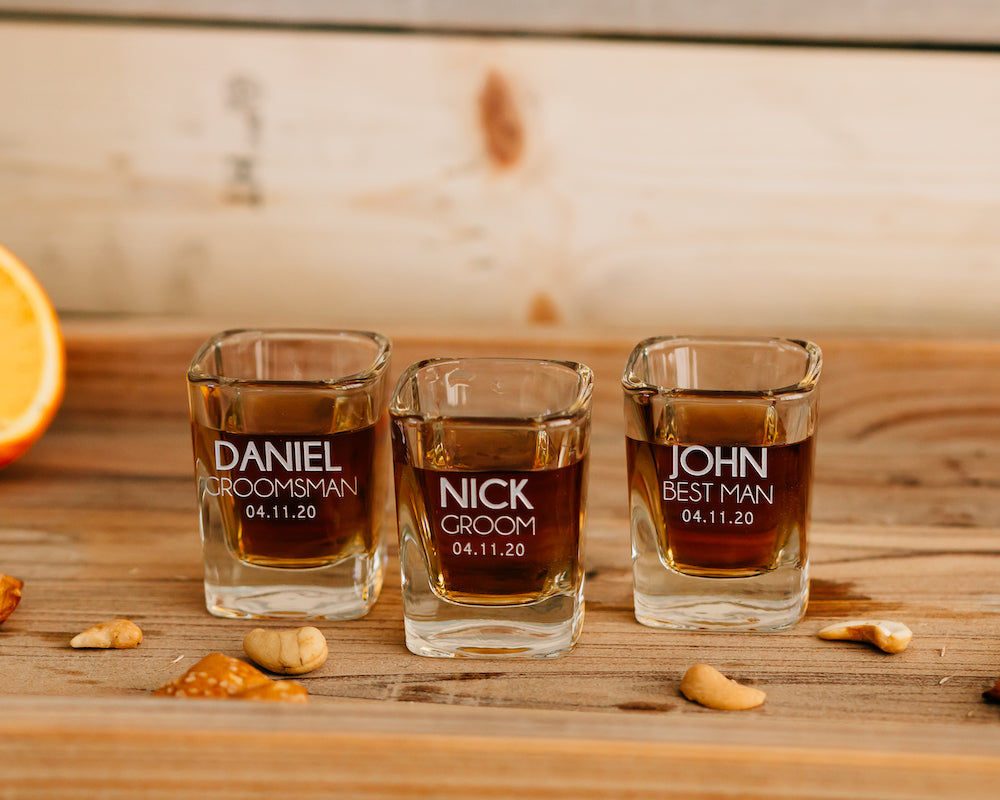The image captures a close-up of three identical square shot glasses with thick bases, neatly arranged side by side on a wooden surface, showcasing the detailed wood grain. Each glass features bold white text; the one on the left reads "DANIEL" with "Groomsman" and the date "04-11-20" beneath it. The center glass displays "NICK" with "Groom" and "04-11-20" underneath, while the right glass says "JOHN" with "Best Man" and the same date. The shot glasses contain a dark amber liquid, possibly whiskey. Scattered around the glasses are brown pretzels and cashew nuts. On the left edge of the image, there's a visible segment of a sliced orange. The wooden backdrop varies slightly in color, presenting a harmonious contrast that frames the shot glasses elegantly.